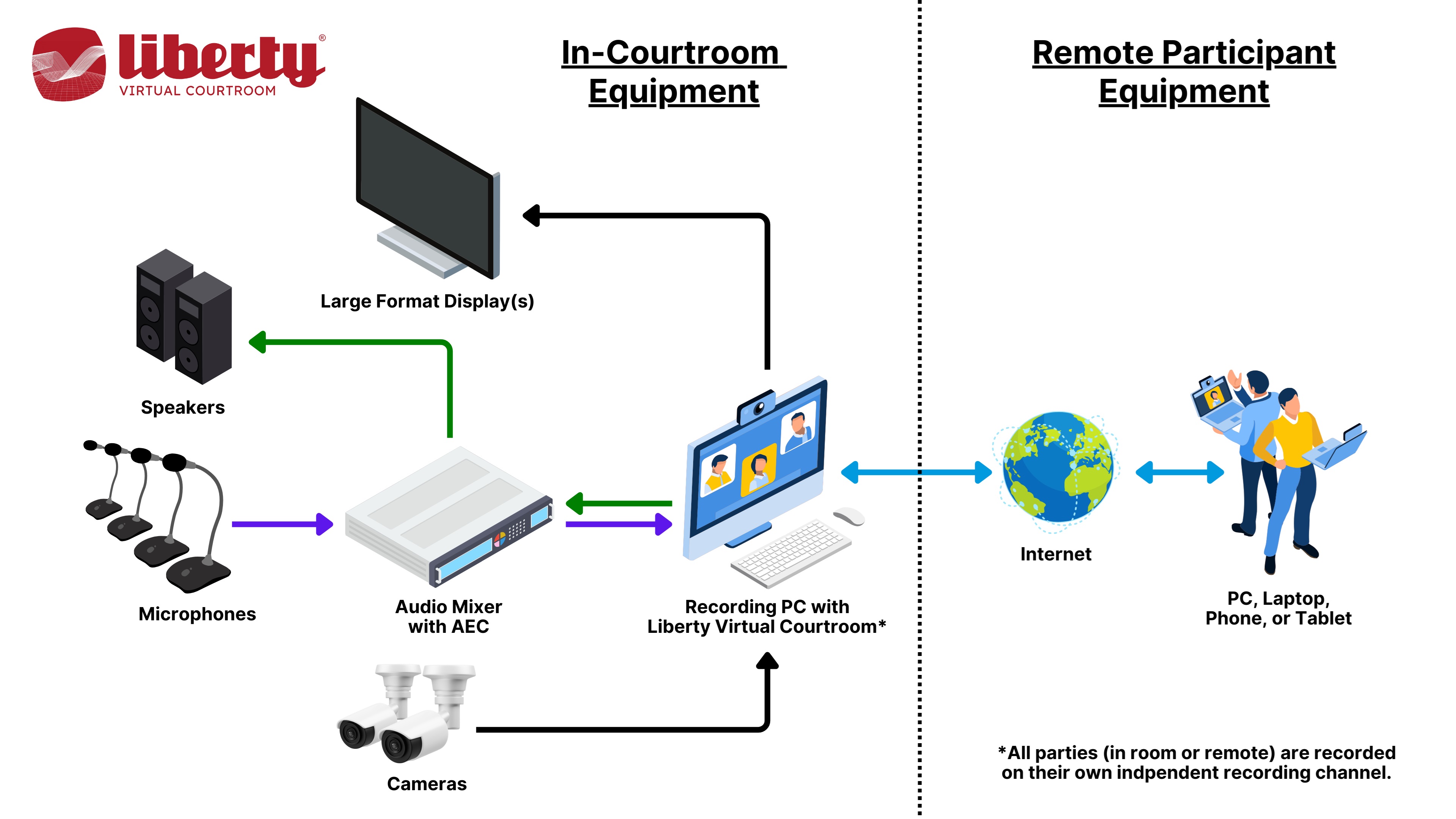The image is an informational chart designed for educational purposes. It features a white background with a thin tan border that has rounded corners, surrounding the entire rectangular image. The top and bottom edges are twice as long as the left and right sides. At the top center, it reads "Liberty Hybrid Hearings" in red text. Below this, on the top left, there are graphics resembling volume knobs and controls labeled "courtroom sound system, DSP." Arrows connect these graphics to an image of a computer screen, labeled "recording and conference PC." Further arrows link this screen to three icons of people denoted as "internet-based remote participants," with an asterisk explaining that these participants, along with all others, are captured in their own audio recording channels. The chart also includes images of microphones labeled "courtroom microphones," connected by arrows to the courtroom sound system. Additionally, it shows three CCTV cameras labeled "courtroom cameras," linked by arrows to the recording and conference PC.